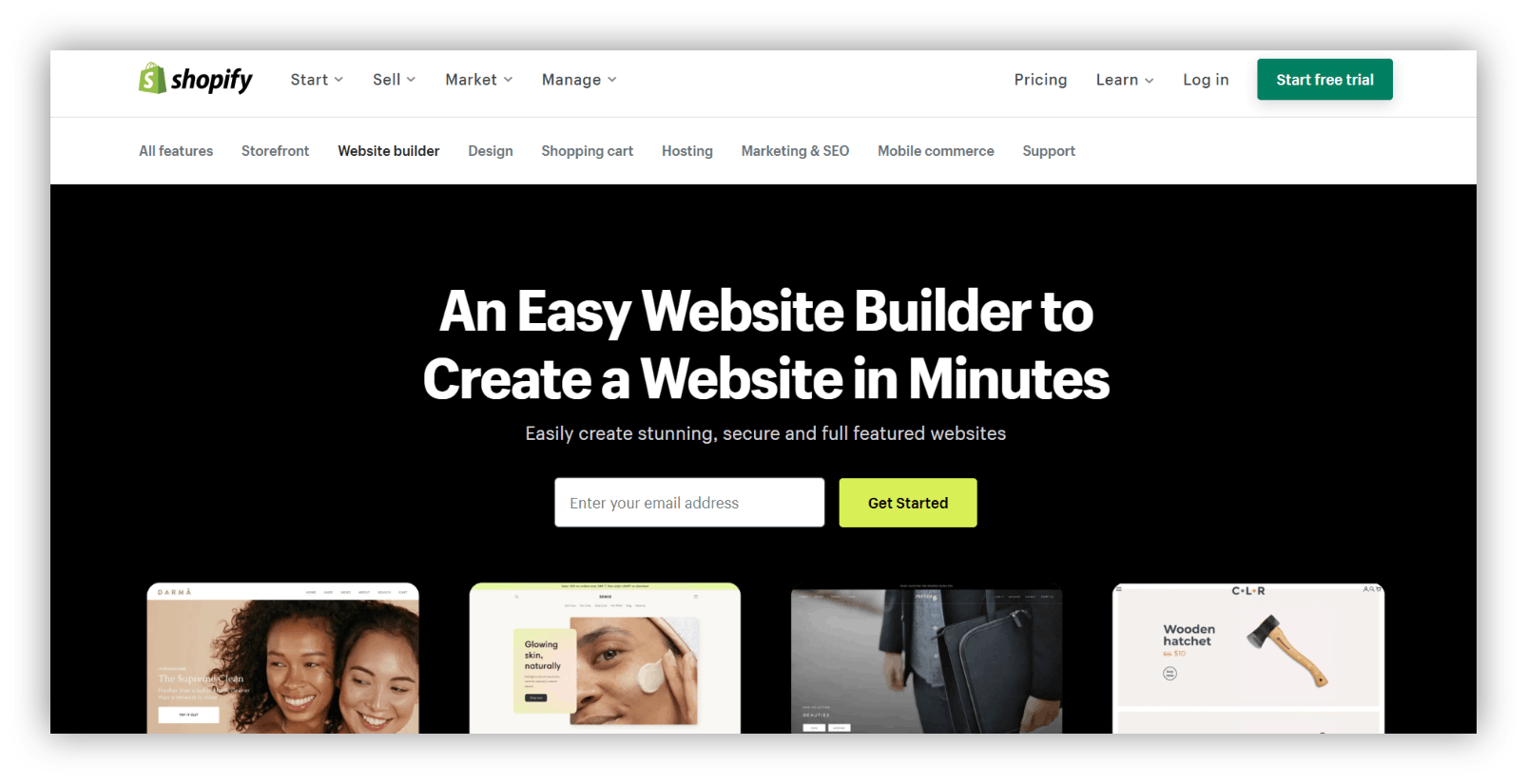The image depicts a Shopify webpage designed for creating and managing online stores. At the top, a green cowbell icon featuring an "S" logo is visible. Directly beneath, the website emphasizes its workflow with steps labeled "Start," "Sell," "Market," and "Manage," each accompanied by downward arrows. 

On the right-hand side of the page, options for "Pricing," "Learn," "Login," and "Start Free Trial" are displayed. Running across the top of the page against a white border are various categories in bold black text: "All Features," "Storefront," "Website Builder," "Design," "Shopping Cart," "Hosting," "Marketing," "SEO," "Mobile Commerce," and "Support."

Directly below, within a prominent black section, there's a bold white headline stating, "An easy website builder to create a website in minutes." The subtext further elaborates: "Easily create stunning, secure, and full-featured websites." Below this informative section, an email address entry field is placed within a white bar, accompanied by a yellow "Get Started" button to encourage user engagement.

The lower segment of the image showcases four pictures. The first image displays two women smiling together. The second image features a woman with an item, possibly makeup, on her cheek, which she's holding with her hand. The third image presents a woman walking with a briefcase slung over her left shoulder. The final image depicts a product: a wooden hatchet, labeled accordingly.